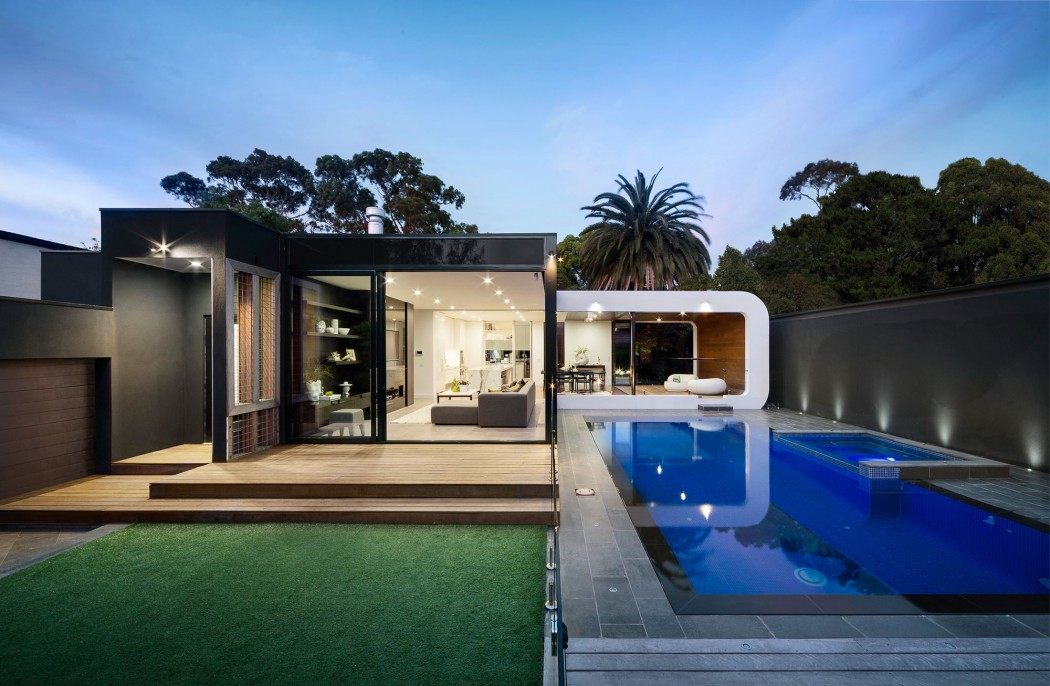This photograph captures a luxurious, modern home with a striking architectural design. The home's exterior is characterized by a sleek black metallic sheen and expansive glass windows, offering a glimpse into a stylish interior featuring a gray sofa, black bookcases, and white shelving. The left side of the image presents a lush, artificial-looking green lawn leading up to a wooden deck that connects to the house's large glass opening. To the right of the house, a deep blue pool extends along the length of the image, framed by a black surround and gray tiling. Adjacent to the pool is a white-walled patio area with wooden accents, featuring two white chairs and a black table. In the background, a white, U-shaped cabana reflects in the pool's serene water. Completing this picturesque setting are blue skies with scattered clouds and towering trees that frame the scene, enhancing the modern elegance of the property.